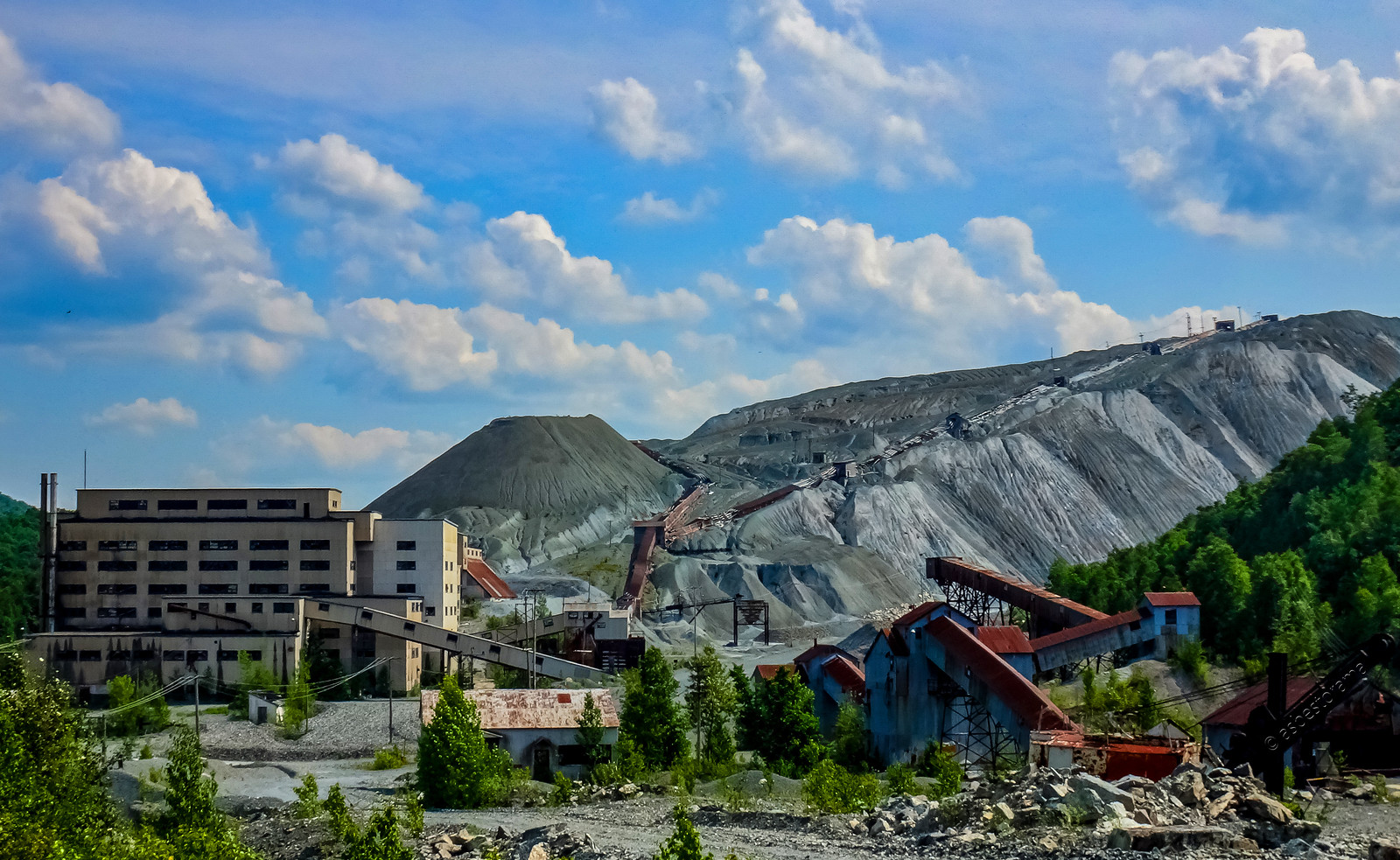The image depicts a large, multi-story industrial complex situated against the side of a gray, rocky mountain. This complex, which features a prominently tan building with several layers and thin, rectangular windows, appears to have seen extensive mining activity. Various chutes and machines indicate active excavation, leading to a landscape marked by piles of rocks and evidence of environmental devastation.

In the foreground, there's a poorly maintained parking lot, hinting at abandonment or neglect. To the right of the main building, there are additional structures, including blue buildings with red roofs showing signs of disrepair, and another smaller building nestled among green trees and rocky cliffs. The sky overhead is blue, dotted with big, fluffy clouds, adding a stark contrast to the man-made and natural chaos below. The scene is framed by scattered pine trees and hints of greenery, which juxtapose the industrial desolation.